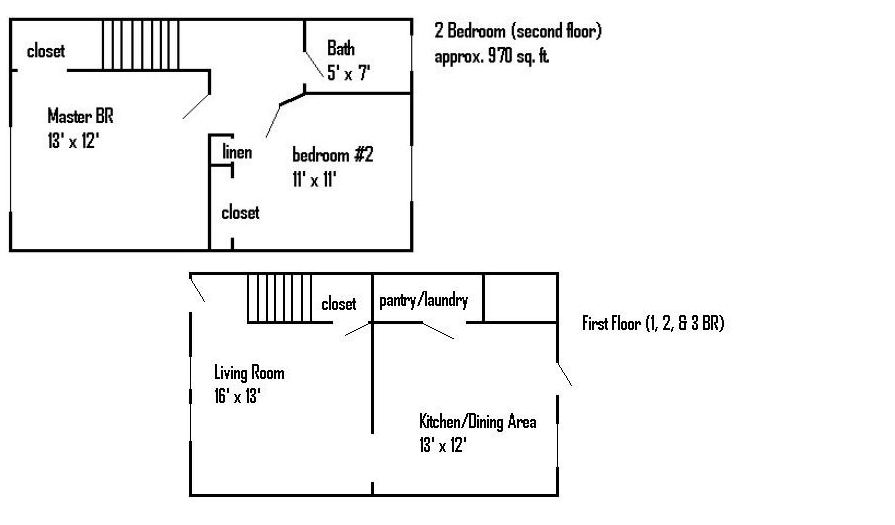Here is a detailed caption for the architect's rendering:

---

This architect's rendering showcases the layout of a two-story house, detailing both the first and second floors. The second floor is represented by a rectangular shape labeled "Two Bedrooms (Second Floor), Approximately 970 Square Feet." At the top of this rectangle, a closet is depicted adjacent to a series of vertical lines indicating the staircase leading downstairs. Within this upstairs area, the master bedroom measures 13 feet by 12 feet, and includes a 5 feet by 7 feet bathroom. The second bedroom, which measures 11 feet by 11 feet, is accompanied by a small closet and a linen closet.

The first floor, represented by the rectangle beneath, is labeled "First Floor, One, Two, and Three Bedrooms." This floor plan is divided into two primary areas: a spacious living room on the left, measuring 16 feet by 13 feet, and an open kitchen and dining area on the right, measuring 13 feet by 12 feet. At the top of this rectangle, a closet is situated next to the staircase. Additionally, the kitchen area at the top includes a pantry and a laundry space, depicted next to an empty square.

---